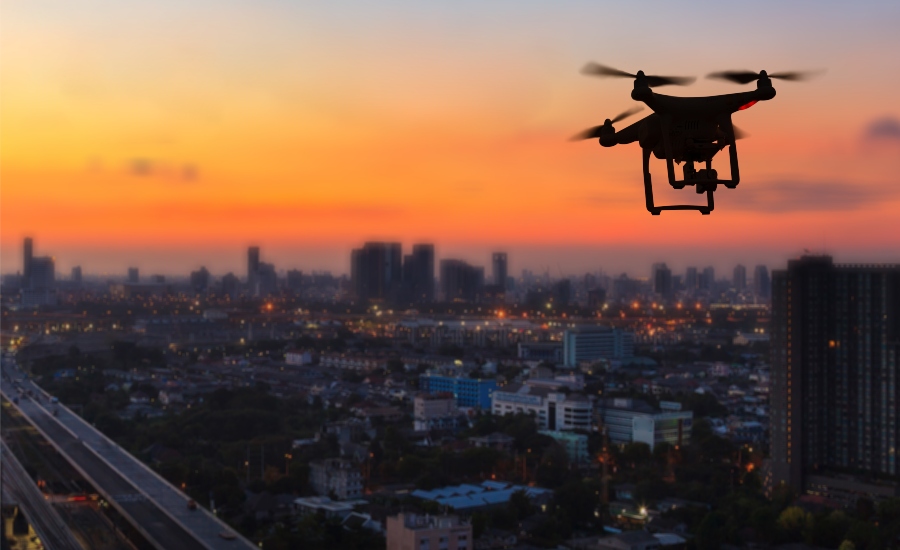This is a landscape-oriented color photograph captured from a high vantage point in the evening. The sky is adorned with a striking sunset, featuring bands of purple, orange, and a golden glow. In the top right corner, a silhouetted black drone with visible propellers and a distinctive red light on its right side hovers high above. Below, the cityscape sprawls out with a mix of illuminated and darkened buildings. Prominently, a skyline of skyscrapers marks the horizon, while several other commercial and residential buildings cluster in the foreground. To the left, a four-lane highway extends diagonally, dotted with cars. The city is alive with various lights, including traffic lights casting red and green hues, contributing to the evening's bustling ambiance.